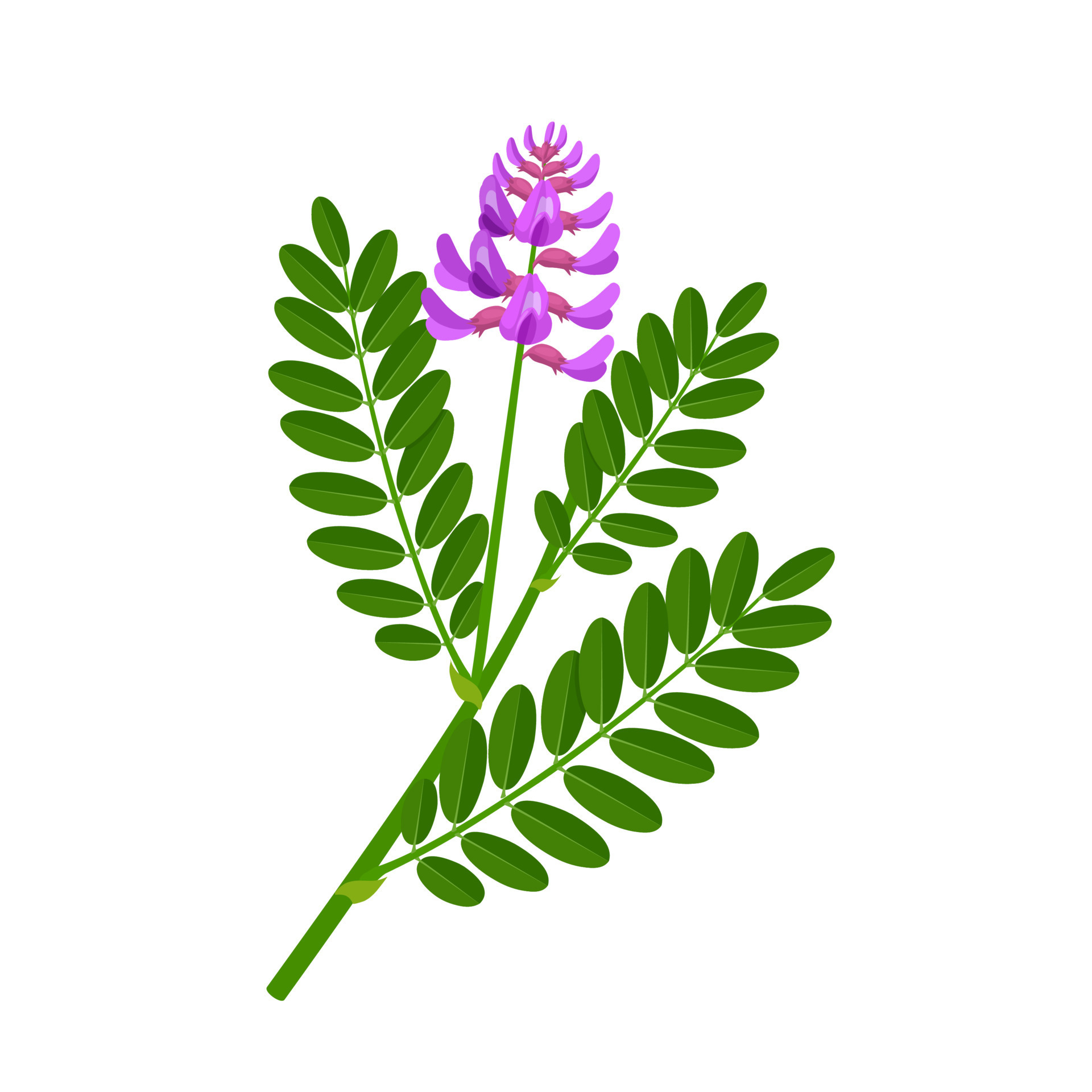The image portrays a botanical drawing of a flowering plant on a solid white background. This plant features a singular, delicate, and slender flower with bright purple, lily-like petals tinged with dark red at their bases. The flower emerges from a green shoot, situated between clusters of green, somewhat oval-shaped leaves with rounded edges. The stem supports three groups of these leaves: the largest cluster is at the bottom right, a medium-sized one is on the left, and a smaller group extends from a small branch. Each cluster consists of opposite leaves. The overall arrangement and elegance of the plant evoke a sense of natural beauty, reminiscent of a plant that would thrive in a southern garden.